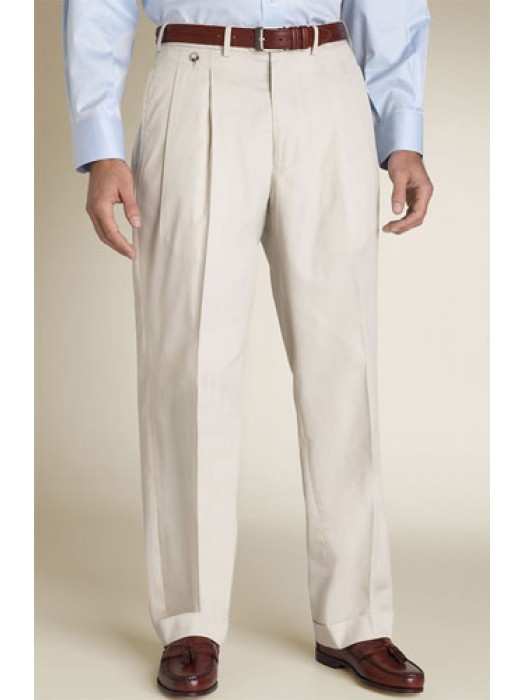The image features a Caucasian male model standing against a tan backdrop, cut off at the waist to only show his legs and lower torso. The man is advertising a pair of light tan, khaki-colored dress pants that are slightly creased, giving them a business casual look. He is wearing a light blue button-down shirt with long sleeves and buttoned cuffs, partially visible. The model sports a thin brown leather belt with a silver clasp, perfectly matching his brown leather loafers, which feature tassels on top. His stance is casual, with his legs straight and arms resting naturally by his sides. The pants fit well, covering the shoes without riding up. The model's left foot is slightly angled, and there is a faint shadow cast behind him on the backdrop. The image emphasizes the fit and style of the formal pants in a business casual context.